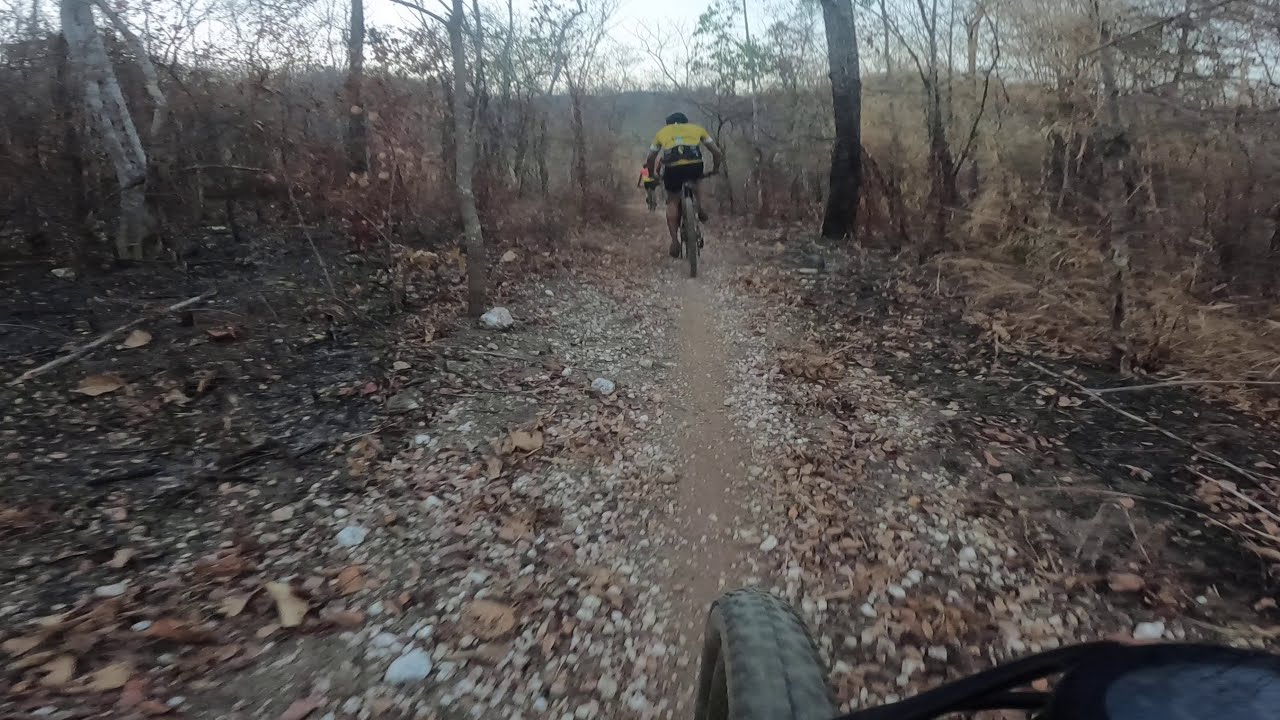In this detailed image, we see a group of three bicyclists navigating a narrow dirt trail through a dense, somewhat desolate forest with hints of past burn marks. The photo, captured from a GoPro likely mounted on the handlebars of a bike, prominently features a rider in a yellow jacket and black shorts with a helmet, positioned in the foreground. Just ahead, another cyclist in an orange shirt is partially visible. The trail is tightly bordered by rocks, leaves, and dead plants, suggesting a challenging ride. The surrounding environment is characterized by a mix of browns, grays, and blacks, with sparse yellow leaves and bare tree trunks, lending an eerie feel to the scene. The overcast sky, barely discernible through the thick canopy, casts a subdued light on the landscape. To the lower right, part of another vehicle, possibly a four-wheeler, edges into the frame, adding to the dynamic and adventurous atmosphere of the ride through what appears to be a remote, rugged terrain.